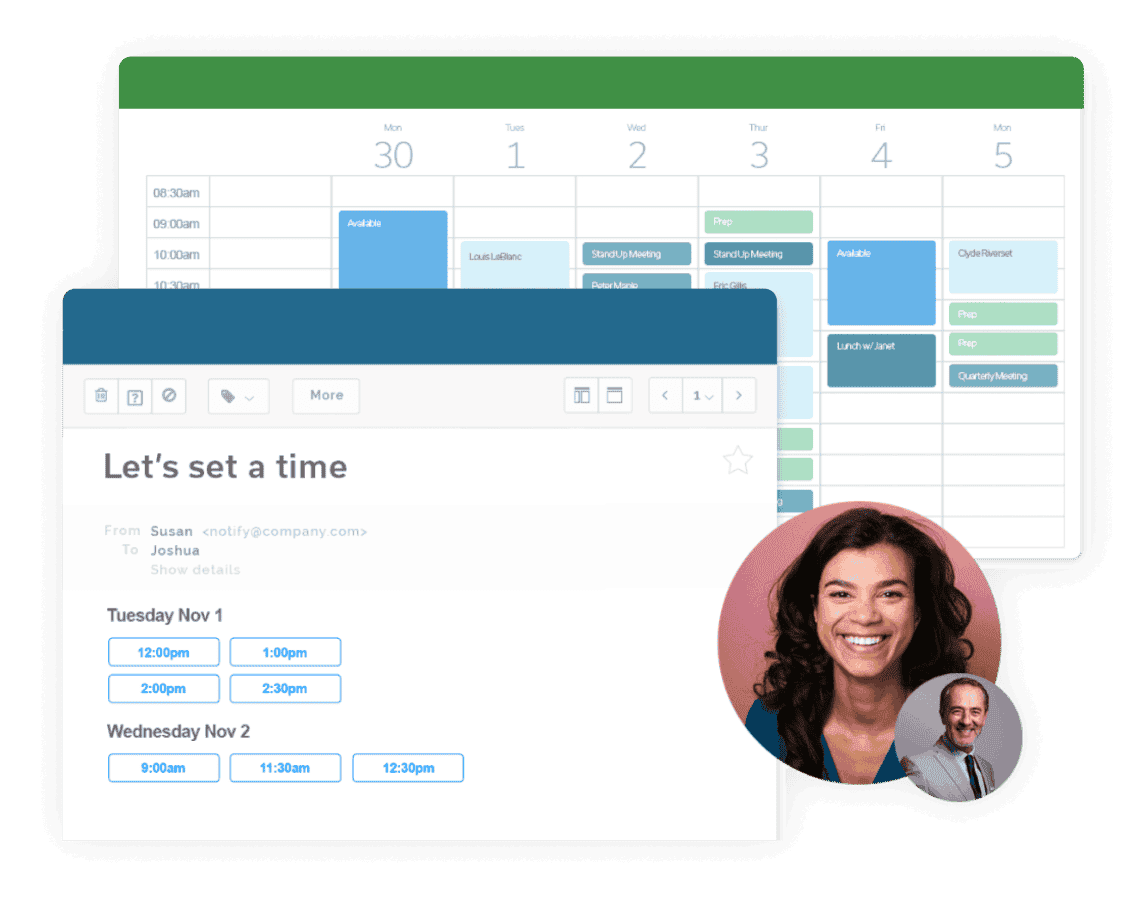The image displays an email invitation template from Susan at notify@company.com to Joshua, requesting to schedule a meeting. The template features a blue header with the text "Let's Set Up a Time" in black letters. Available time slots for the meeting are listed as follows: 

- Tuesday, November 1st at 12:00 PM, 1:00 PM, 2:00 PM, and 2:30 PM.
- Wednesday, November 2nd at 9:00 AM, 11:30 AM, and 12:30 PM.

The dates and days are written in black, while the times are highlighted in blue. To the side, a large circular photo of a woman (presumably Susan) next to a smaller circular photo of a man (presumably Joshua) are displayed. Behind the email invitation, a calendar is visible, showing a week's schedule color-coded in blue and green with half-hour increments. The view is partially obscured by the invitation, but it shows the dates from Monday, October 30th to Monday, November 5th, with an available slot on Wednesday, November 2nd at 9:00 AM suggested as the best option for the meeting.